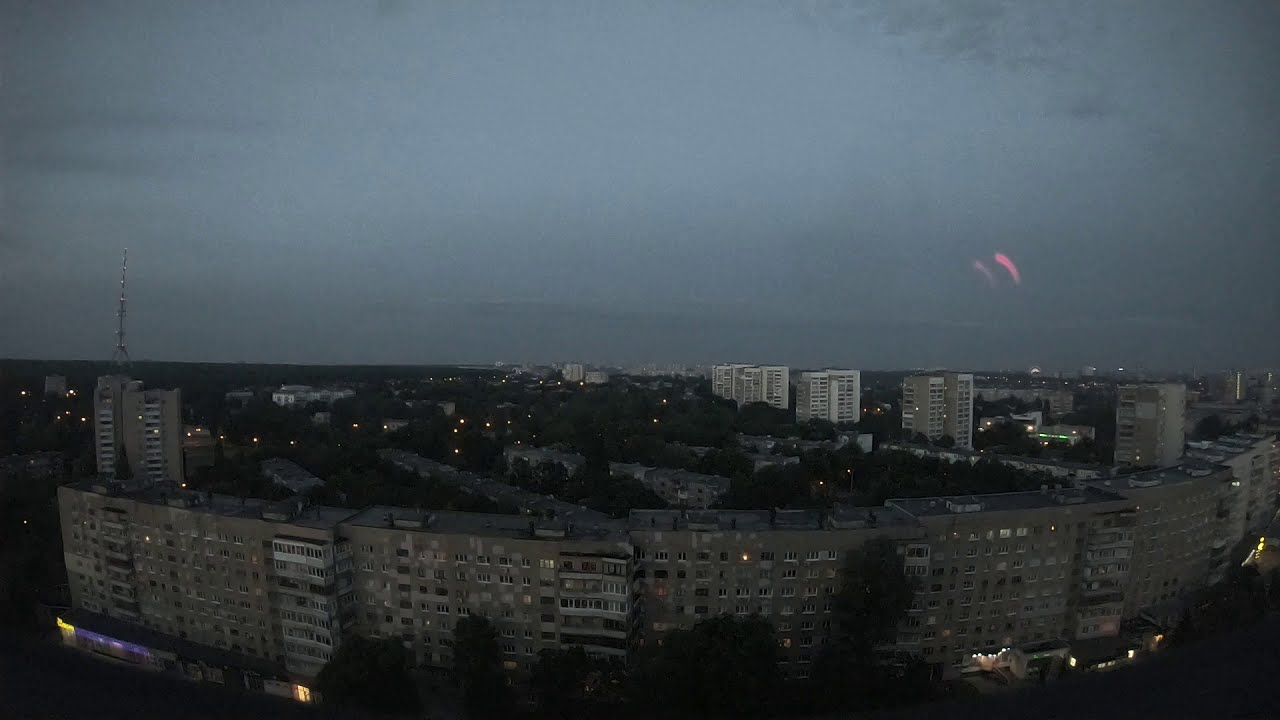In this evening-to-night photograph of a city, the foreground is dominated by a semi-circular wall of large, gray, and black apartment buildings stretching from the left to the right. These structures are approximately eight to ten floors high and feature dark, unlit windows and wider balcony edges on their right sides, giving them a distinct appearance. The left portions of these buildings are predominantly dark brown. A tall TV-like tower is situated on the left side of the image. 

In front of these buildings, a few trees are visible; however, the majority of the greenery, including a prominent tree toward the center right, is located behind this main wall of buildings among smaller, residential structures. Beyond these, a cluster of white-colored apartment buildings rises in the back right, further contributing to the layered depth of the cityscape. 

The top two-thirds of the image features a darkish blue, cloudy night sky, enhancing the nighttime ambiance. Dotted streetlights can be seen in the bottom right, casting subtle glows that outline the city streets. The scene is devoid of vehicles, reinforcing the stillness of the night.